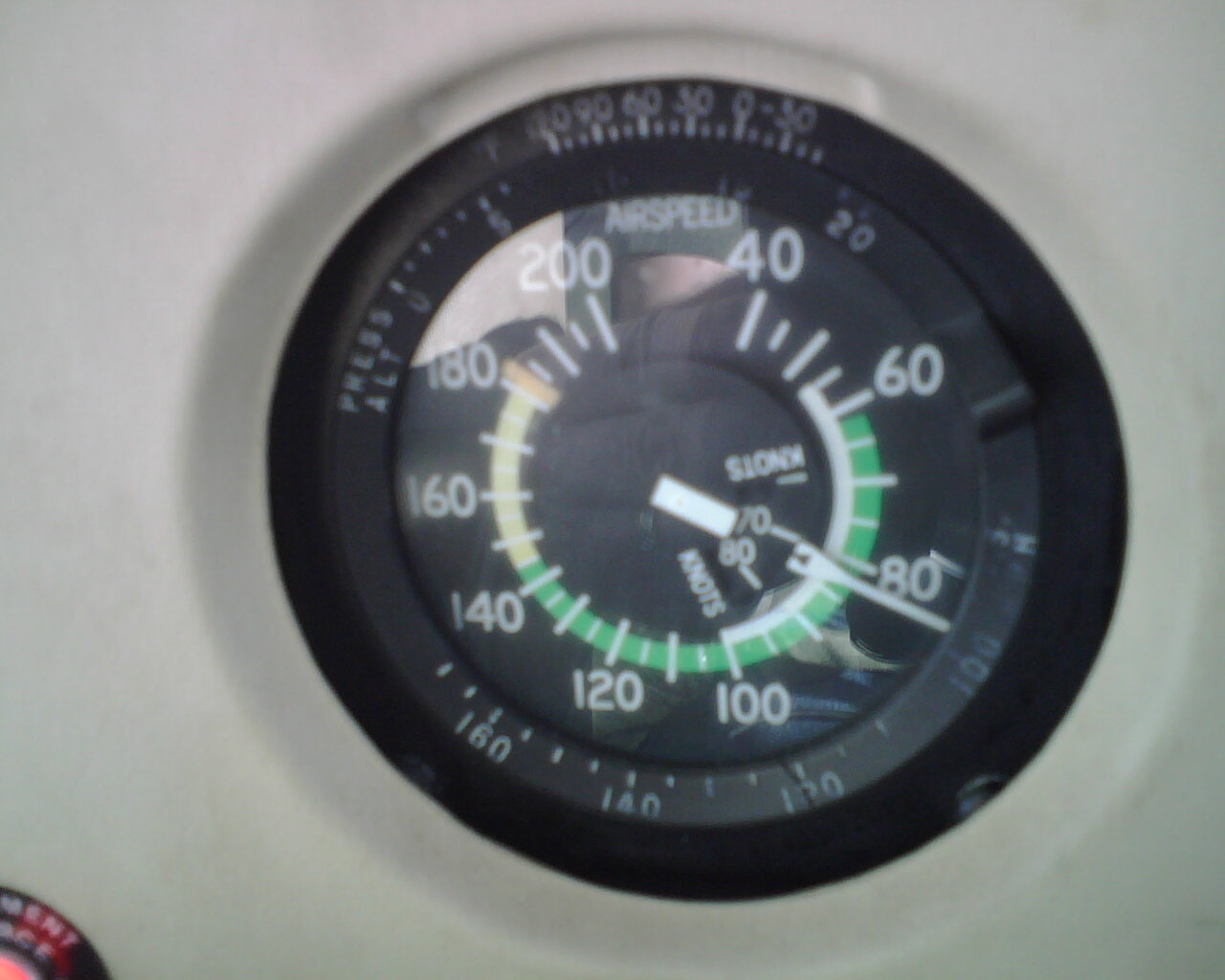This detailed photograph showcases a black mechanical dial set against a stark white background, occupying approximately 70% of the frame and slightly off-center towards the right. The outermost rim of the dial features a series of numbers arranged from right to left, specifically: -30, 0, 30, 60, 90, 120, each accompanied by small notches. 

Moving inward, there is another concentric set of numbers starting from the middle left, labeled "Press Alt", followed by numbers 0, 5, 10, 15, and 20, each with corresponding notches.

The bottom half of the dial continues this numerical progression with markings at 160, 140, 120, and 100, each again highlighted by notches above them. The innermost circle of the dial prominently displays the word "Airspeed" at the top. To the right, another sequence of numbers arcs clockwise: 40, 60, 80, 100, 120, 140, 160, 180, and 200. 

A central needle or indicator is present within the dial, presumably pointing to the current airspeed measurement. This intricately detailed instrument likely serves a critical function in the accurate assessment of airspeed, capturing the essence of precision required in mechanical dials.